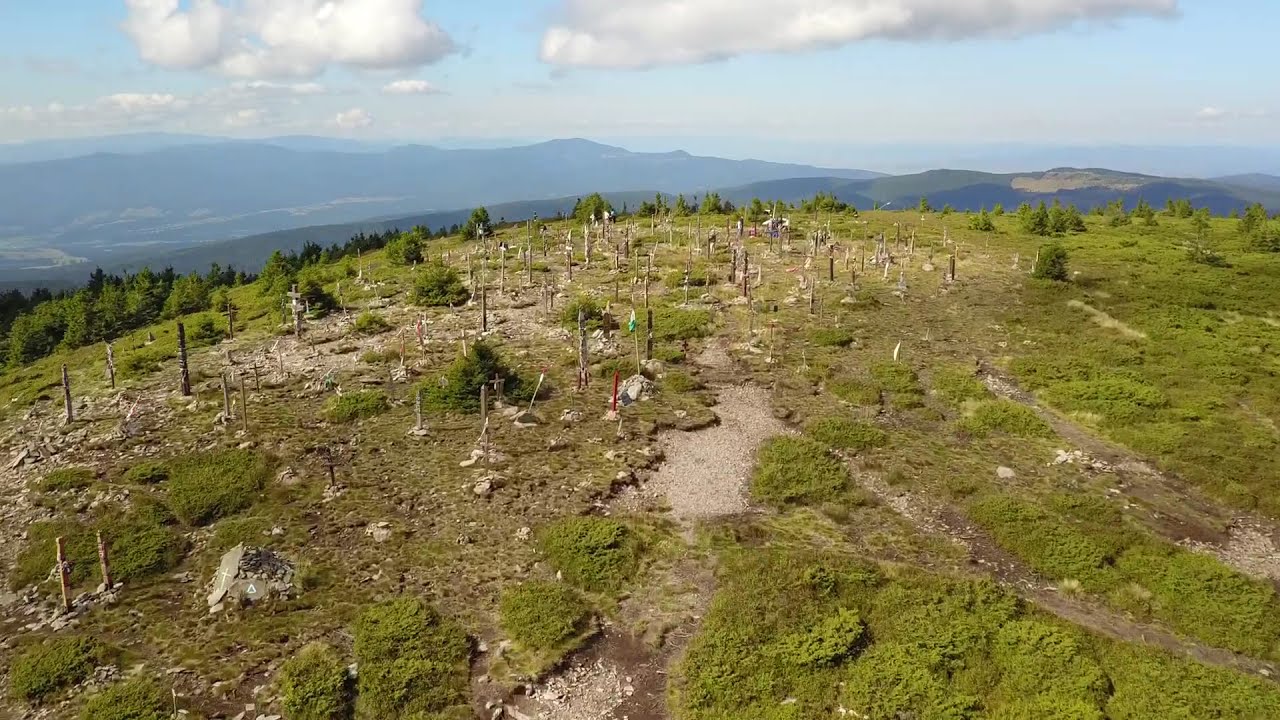The image depicts an aerial view of a remote, natural area resembling a makeshift, primitive graveyard situated on the side of a hill. The ground is scattered with a multitude of sticks and wooden poles, some of which resemble crosses and totem poles, suggesting grave markers. These markers are often surrounded by small mounds of rocks. The terrain is largely brownish, punctuated by patches of gravel, stones, and low-lying shrubs or moss.

In the foreground and middle ground, the landscape is dominated by rocky surfaces and patchy grass, with occasional clumps of bushes and shrubbery. The background reveals a range of misty mountains and an assortment of darker green evergreens and taller trees, adding depth to the scene.

The sky above is a gradient of light to darker blues, with several large clouds ranging from white to darker gray, creating an atmospheric effect. The sky and mountainous horizon occupy about one-third of the image, while the rugged, grave-marked terrain takes up the remaining two-thirds. The overall scene evokes a sense of solemnity and ancient tradition in a strikingly raw and natural setting.